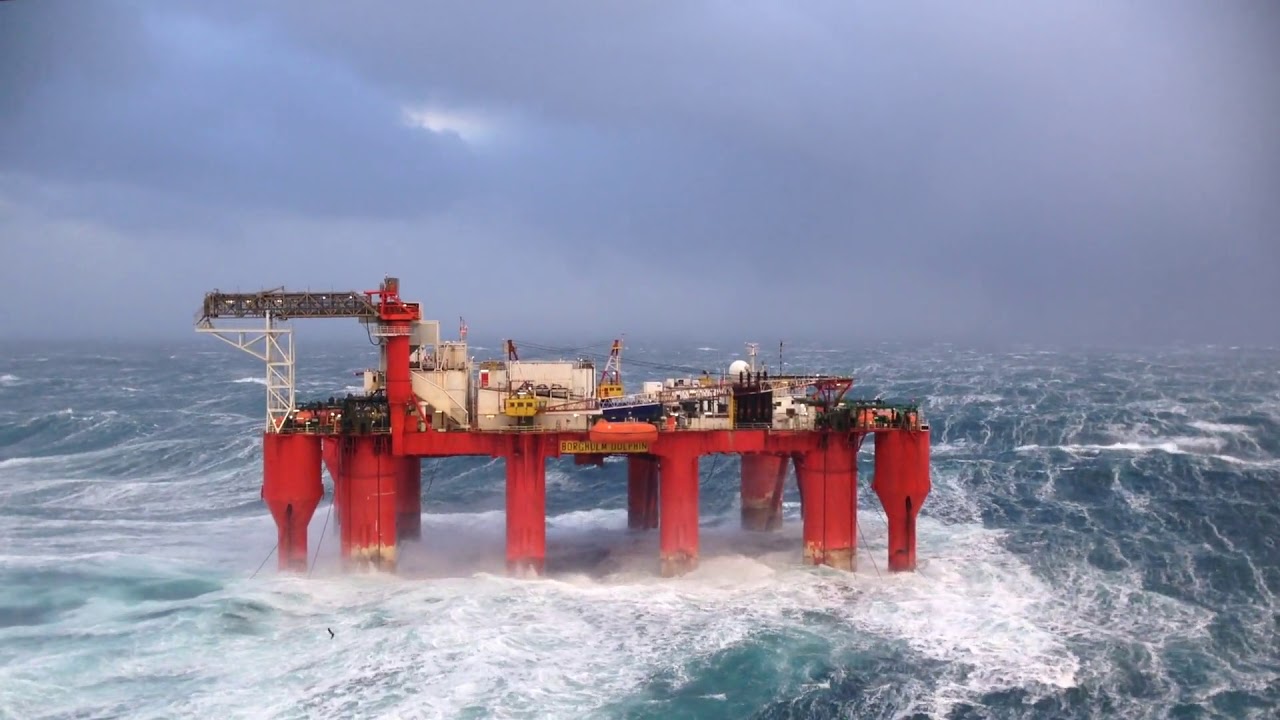This detailed photograph captures an offshore oil rig weathering a fierce storm in the middle of the ocean. Central to the image is the rig, supported by a series of ten bright red pylons or columns that plunge into the rough, foamy water below. The rig’s upper structures, predominantly colored in white or beige, feature various buildings that could serve as sleeping quarters or workspaces. Yellow cranes are scattered across the platform, with one particularly noticeable on the left side. The sky is ominously dark and cloudy, almost blending with the turbulent blue ocean. A faint glimmer of light breaks through the clouds on the center-left side of the image. Towards the bottom left corner, a crane extends outward, with cables or chains descending from it into the water. Notably, there are three individuals clad in orange rain suits visible on the lower left side, adding a human element to this dramatic scene. The photo appears to have been taken from a helicopter, providing an expansive view of the ocean stretching endlessly to the horizon without any visible landmasses.